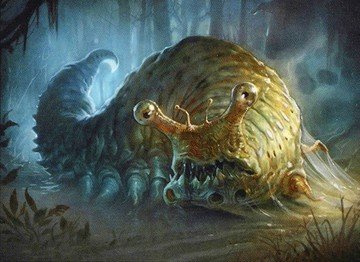The image is a detailed, full-color artistic piece with a square frame and no specific border or background. In the lower left and right corners, there is noticeable vegetation, while the upper left has some vegetation alongside grayish tree trunks. The upper right features a white area resembling a ghost face with two large black eyes and a black mouth. The central focus of the piece is a grotesque, slug-like monster, primarily brown with hints of gold, yellow, and dark gray. This creature has a long body with numerous legs that extend back to a tail. It has beady eyes on stalks with some antennae underneath and a mouth open wide, revealing teeth. The monster is positioned centrally and appears to be looking directly at the viewer. It is laying on dirt, and the depiction of the setting is somewhat ambiguous—possibly resembling a cavernous environment. The overall style suggests a digital print or a meticulously painted or drawn image, but it is unclear whether it’s the result of an artist's handwork or a software application.